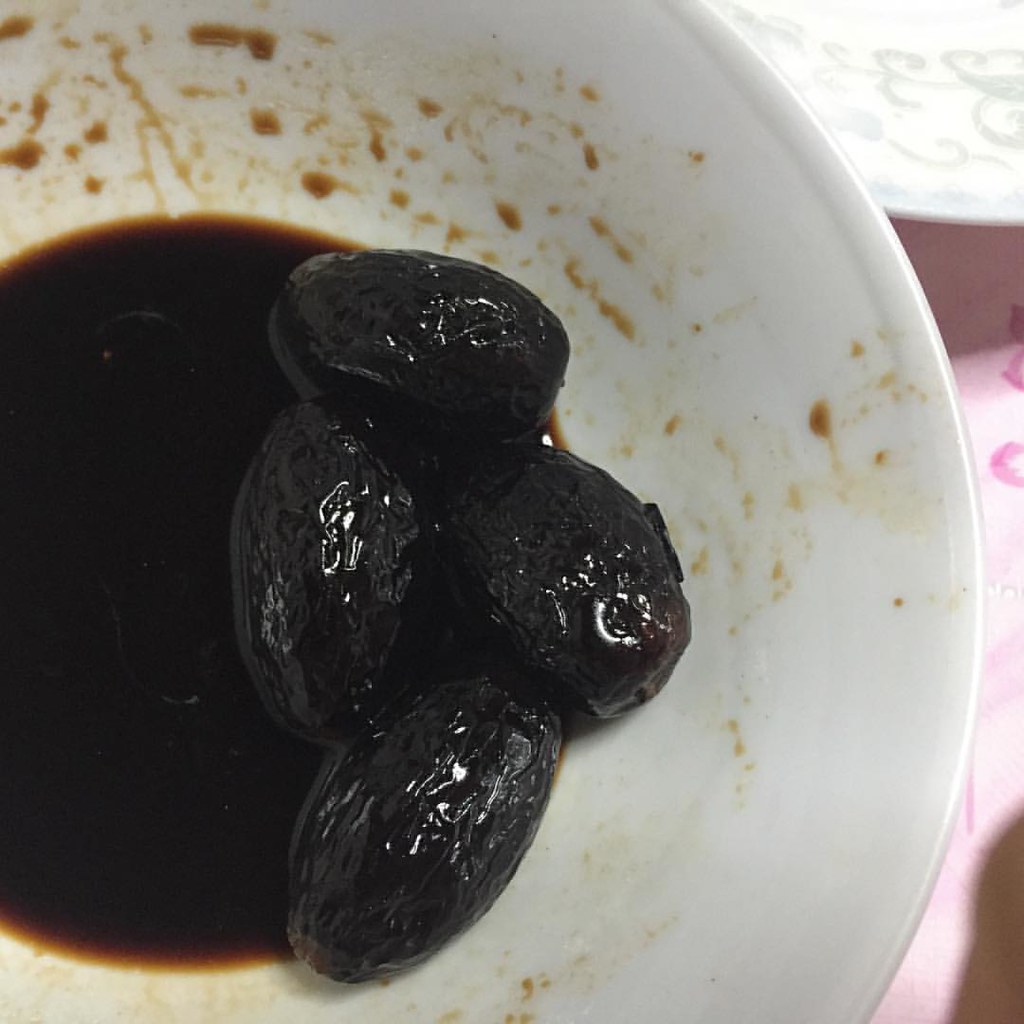In the image, a large, white porcelain bowl dominates the frame, filled with a dark brown liquid resembling coffee. Four oblong, wrinkled fruits, likely prunes, sit immersed in this liquid, which is pooled at the bottom and has splashed up along the sides, leaving streaks behind. The prunes, dark and shiny, with reflections of white light, have likely released their juices into the liquid. The background features a white tile in the upper right corner and a partially visible white plate adorned with light blue designs and a blue rim. The scene is set on a tablecloth that is predominantly white but patterned with small pink hearts and flowers.